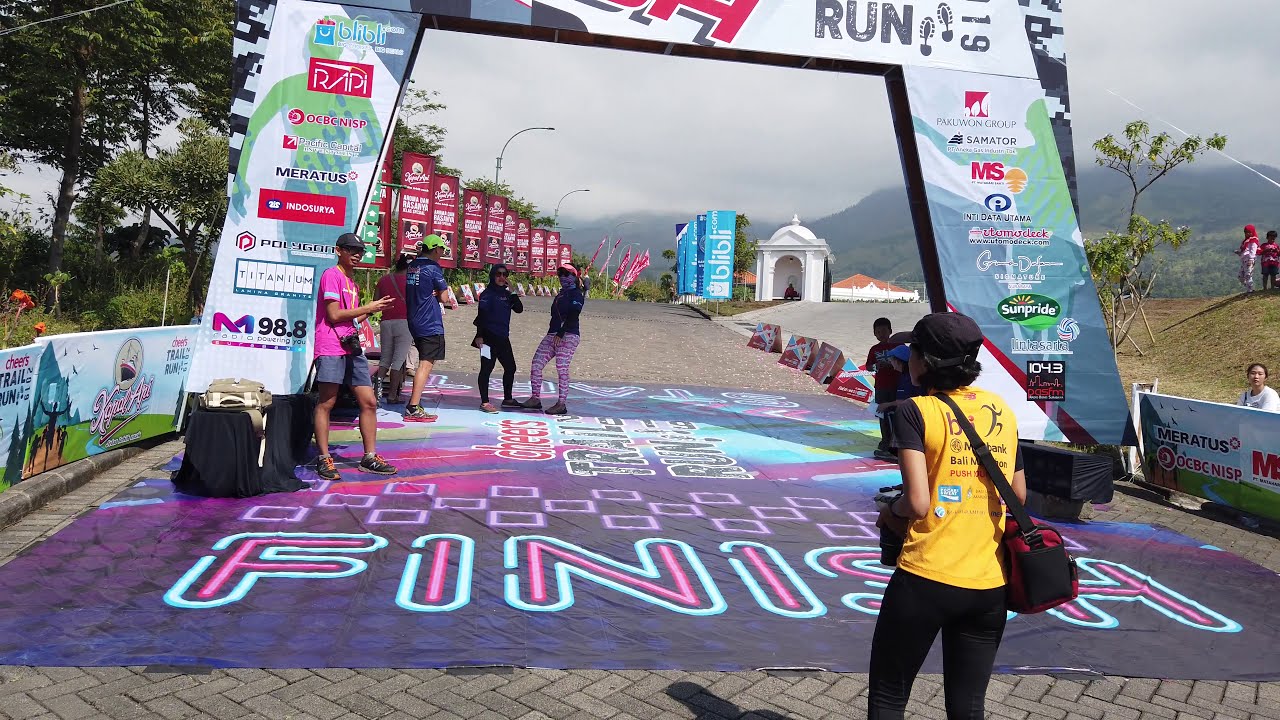The photograph captures a vibrant and bustling scene at the finish line of a race, taken outdoors during the daytime. We're positioned behind a female runner who has just crossed the finish line. She is dressed in a black ball cap, a yellow shirt with black short sleeves, black running pants, and is carrying a red handbag with a shoulder strap. The wide, brick-paved walkway beneath her can accommodate 10 to 12 people shoulder to shoulder.

Prominently featured is an elaborate archway marking the finish line, adorned with numerous sponsor logos including "Maratos," "Sun Pride," and a radio station "98.8." The word "FINISH" is displayed on the ground in bright pink neon lettering outlined in black and surrounded by a neon blue border. The archway itself, resembling a trapezoid with angled supports, stands over a wide stone street. Behind the arch, a white gazebo-like structure is visible against a backdrop of trees and distant mountains. Spectators can be seen standing under the arch, some looking towards us, possibly cheering and waiting for more runners to cross the line. The image is rich with color and detail, capturing the energy and community spirit of the event.